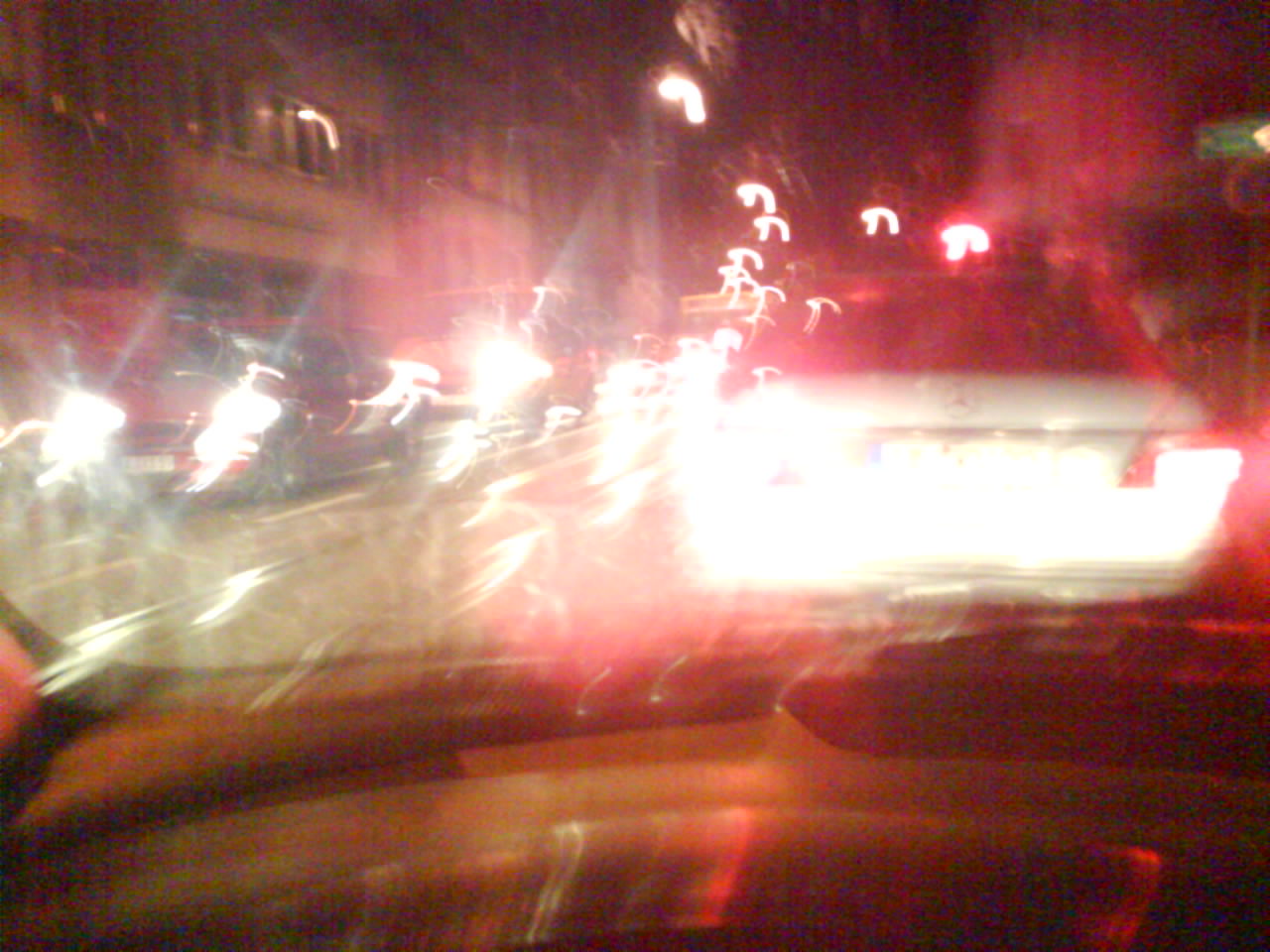This photograph captures an extraordinarily blurry nighttime scene taken from inside a moving vehicle, looking out through the front windshield. The image is full of visual noise and streaks, likely due to the car being in motion when the picture was snapped. The scene is illuminated by several streetlights, which create stretched, horseshoe-shaped glares across the photograph. In the lower part of the picture, the car's dashboard is faintly visible in gray-black tones, reflecting some of the lights in red and white.

To the left, dimly discernible buildings, possibly apartments with off-white windows, provide a backdrop. The vehicle directly ahead has its taillights on and appears to be white with a black top. On the opposing side of the road, approaching cars form blurred streaks of light; one of them, a red truck, stands out in the middle-left section of the image. The overall effect is chaotic, with various red and white streaky lights punctuating the dark, blurry scene.